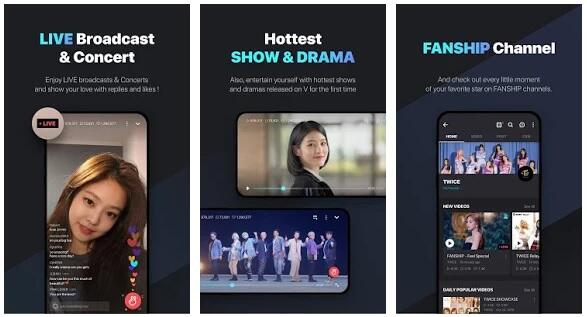The image features a monochromatic black background divided into three equally sized vertical sections.

**Left Section:**
- **Headline:** "Live Broadcast in Concert" in a combination of blue and white text. 
- **Blurry Subtext:** "Enjoy live broadcasting concerts and show your love with replies," with the remaining text being illegible.
- **Visual:** Below the text is an image of a smartphone screen. Displayed on the screen is a young woman with long brown hair past her shoulders, looking towards the camera and smiling. The text on the phone screen is blurry and unreadable.

**Center Section:**
- **Headline:** "Hottest Show in Drama."
- **Blurry Subtext:** "Entertain yourself with the hottest shows and dramas released on," with the remainder presumably cut off, possibly starting with the letter "V."
- **Visual 1:** A phone screen showcases a woman with short dark hair just below her shoulders.
- **Visual 2:** Below this, another phone screen features a group of eight people on stage.

**Right Section:**
- **Headline:** "Fanship Channel."
- **Blurry Subtext:** "Check out every little moment of your favorite star on Fanship Channels."
- **Visual 1:** A phone screen displays a group of around nine women facing forward, dressed in fancy clothing.
- **Visual 2:** Below this, a phone screen shows a woman alone, dressed in a black dress.
- **Additional Visual:** There is a partially visible and unidentifiable image beside the woman in the black dress.

Incorporating these elements, the detailed caption would read:

"An intricately designed image set against a black background, divided into three equal sections. The leftmost section highlights 'Live Broadcast in Concert' with elements in blue and white, and contains a blurred subtext about enjoying live concerts and showing love with replies. A displayed smartphone screen captures a photo of a young woman with long brown hair smiling at the camera, overlaid with indistinct text. The central section promotes the 'Hottest Show in Drama,' encouraging viewers to entertain themselves with trending dramas. Below this, one phone screen shows a woman with short dark hair, while another features a group of eight people on stage. The rightmost section introduces the 'Fanship Channel,' inviting fans to catch every moment of their favorite stars. Here, a phone screen displays a group of around nine elegantly dressed women, complemented below by an image of a woman in a black dress. Another partially visible image adds an element of mystery to this channel's offering."